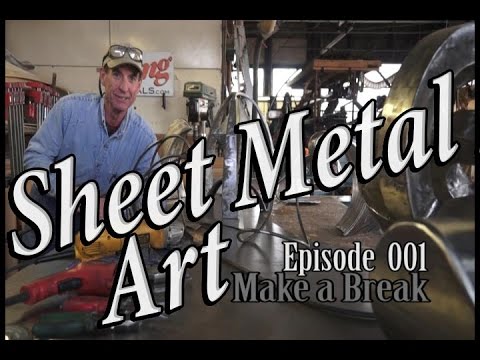The image resembles a title card from a television show. Prominently featured in bold, black-outlined white letters are the words "Sheet Metal Art" followed by "Episode 001" in the same style. Below this, in grey text, it reads "Make a Break." On the left side of the frame, a man stands out distinctly; he wears a khaki-colored baseball cap with safety goggles resting atop it and a long-sleeved denim button-up shirt. His expression is slightly smiling. Behind him, there's a partially visible white sign on a wall, displaying the letters "NG" and "LS.com." The background suggests an industrial setting, with visible machinery, metal objects, a large circular piece, and various tools. A big metal table in front of the man holds several tools, including a red drill and another drill behind it. The overall scene gives the impression of a bustling metal workshop or factory environment.